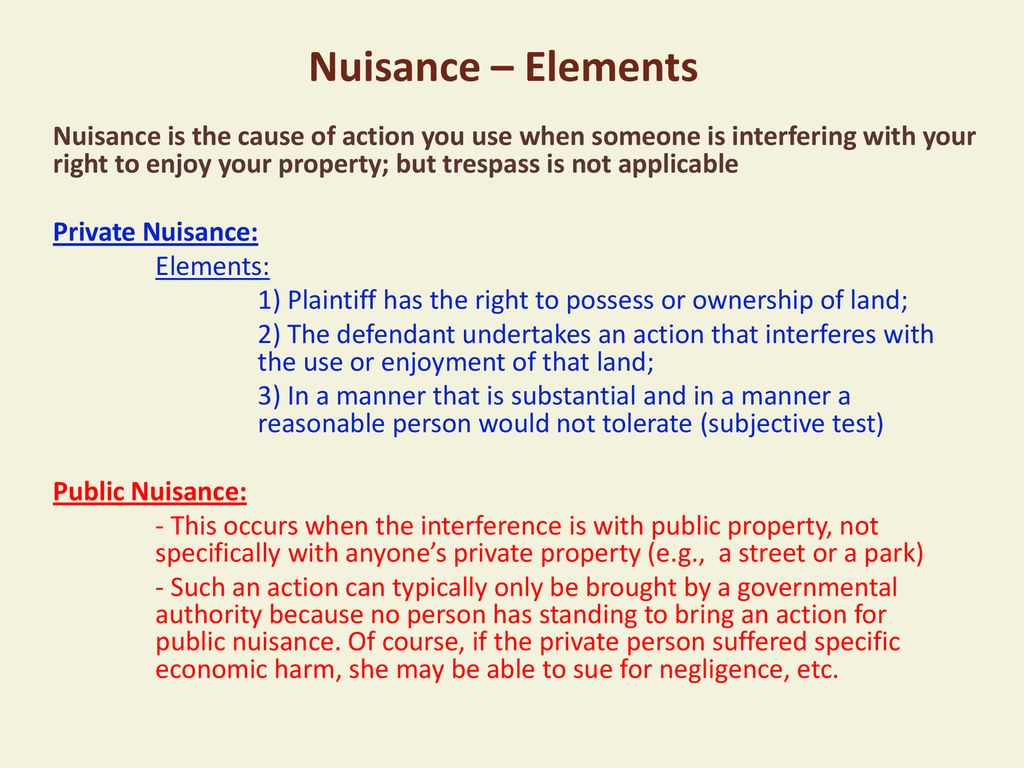The image features an off-white beige background with various sections of text, each in a different color for emphasis. At the top, there is a title in brown text that reads "Nuisance Elements." Directly below, also in brown, is a description stating, "Nuisance is the cause of action you use when someone is interfering with your right to enjoy your property, but trespass is not applicable."

The middle section focuses on "Private Nuisance" and is outlined in blue text. It details the conditions under which a private nuisance is recognized: 1) The plaintiff must have the right to possess or own the land. 2) The defendant must take an action that interferes with the use or enjoyment of the land. 3) The interference must be substantial and intolerable to a reasonable person, which is described as passing a subjective test.

Further down, in red text, the next section is titled "Public Nuisance." This part explains that a public nuisance occurs when there is interference with public property—such as streets or parks—that is not owned by any specific individual. Such actions generally can only be litigated by a governmental authority since individuals do not have standing to call out public nuisances unless they have suffered specific economic harm, in which case they may sue for negligence or other legal reasons.

Overall, the image appears to serve as an informative infographic that outlines legal distinctions and examples related to nuisance law, categorizing nuisances into private and public with detailed explanations and criteria for each.